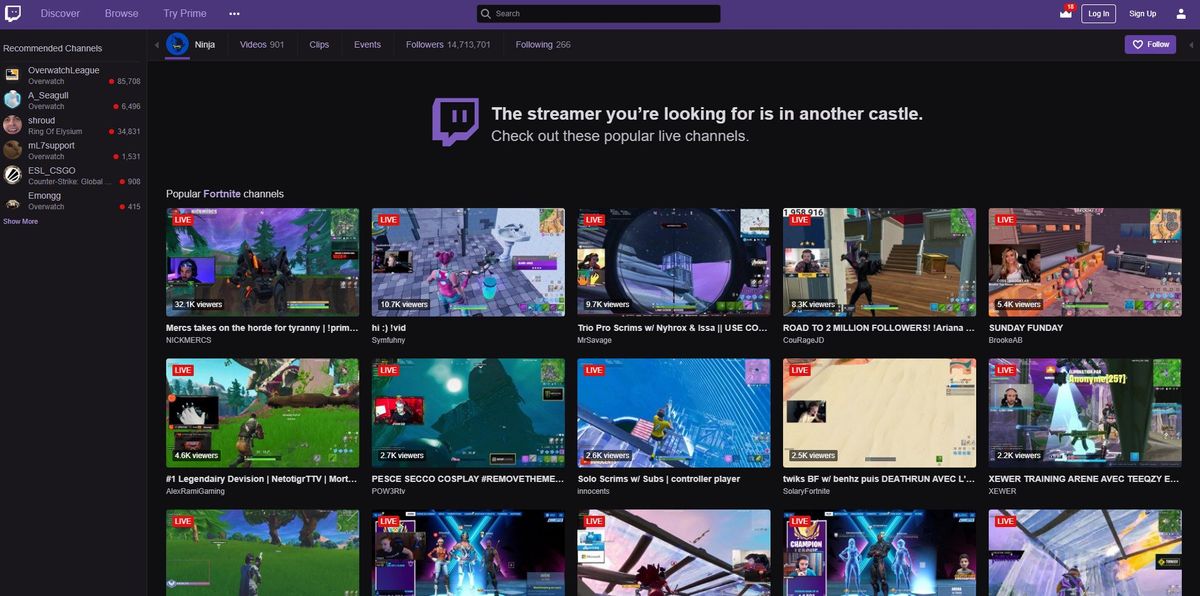The image appears to be a webpage interface, possibly from a computer. At the top, there is a purple search bar accompanied by a chat icon and several clickable options: "Discover," "Browse," and "Try Prime," hinting that this could be an Amazon Prime interface. To the right of these options are three vertical dots, and a search bar. Continuing further to the right, there are icons for notifications, login, sign up, and a user profile, represented by a small person icon.

Below this purple header, there is a sign-in screen, followed by a section featuring 15 icons, which seem to represent different channels. Above these icons, there is a centered message stating, "The streamer you're looking for is in another castle, check out these popular live channels." On the right side of the page, there is a section that likely shows users who are logged into the channel, though it is difficult to see due to the small size of the icons.

The first group of five channels is titled "Popular Fortnite Channels," indicating that all the listed channels are related to Fortnite. These channels are displayed in colorful squares with titles beneath them, suggesting that users can choose one to watch or join. The overall aesthetic of the webpage is vibrant and engaging, designed to attract users to popular live Fortnite streams.